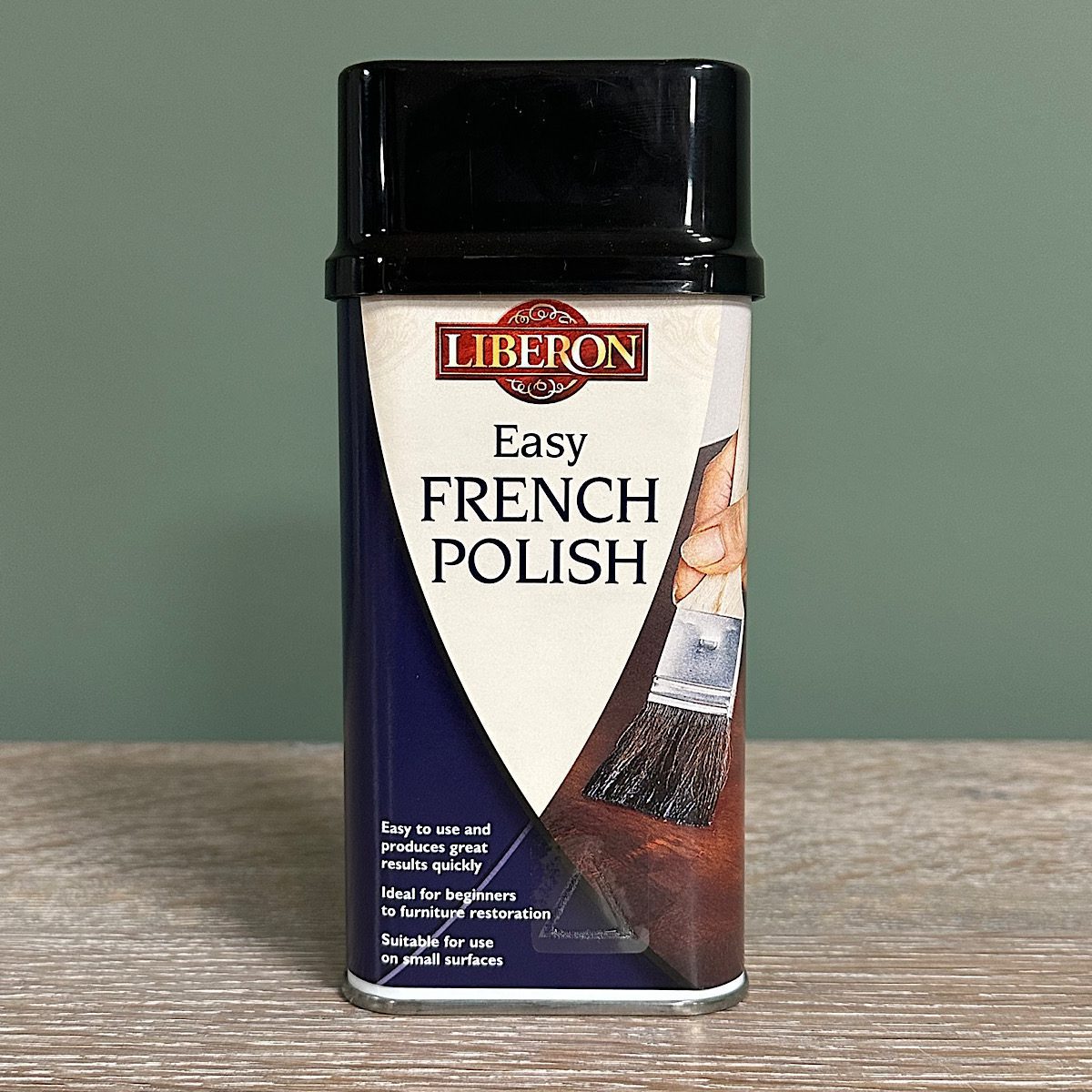This image is a detailed product photograph for a Liberon Easy French Polish, targeted towards furniture restoration enthusiasts. The product is contained in a tall, rectangular metal can with a glossy black, oval cap. The can is predominantly white with distinctive diagonal color bands: a deep blue on the bottom left and a varnish brown on the bottom right. Both streaks converge towards the top, leaving a prominent central area in a beige shield shape.

In bold black text, the center label reads "Easy French Polish." Below this, on the blue-colored streak on the left, white text provides user-friendly details: "Easy to use and produces great results quickly. Ideal for beginners to furniture restoration. Suitable for use on small surfaces."

The brand name, "Liberon," is showcased right under the cap in elegant gold lettering within a red rectangular border that includes a circular accent in the middle. The brown streak on the right features an image of a hand holding a paintbrush, applying the polish to a wooden surface, demonstrating its use.

The can sits on a light brown wooden table, with the background being a contrasting dark green wall. This setting highlights the product as an ideal tool for effortless and effective furniture restoration, perfect for those new to the craft.